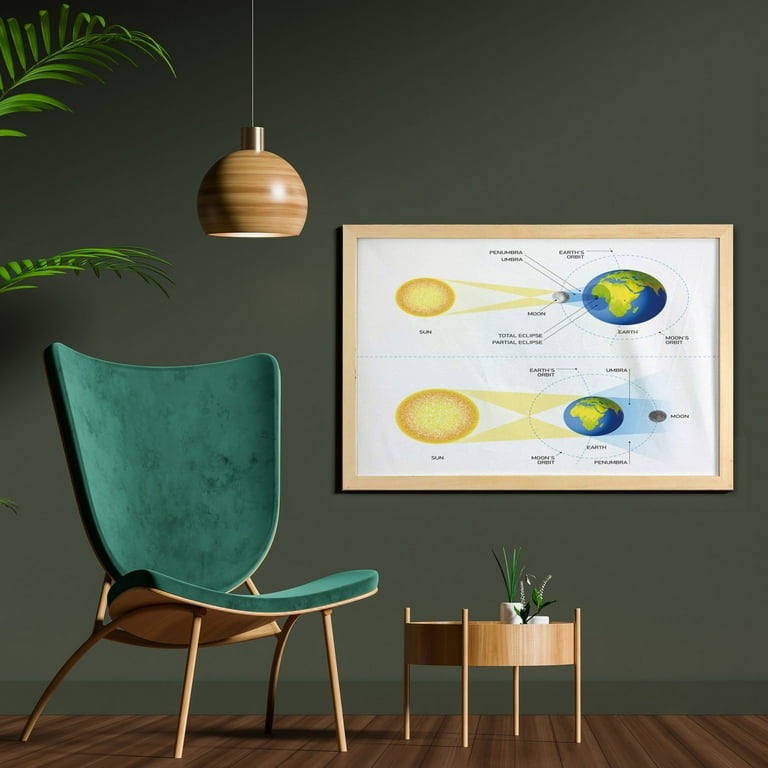This photograph captures a stylish and contemporary small room with a distinct design aesthetic. The room features a wooden floor with visible grain patterns, complementing the gray olive green wall color. In the left corner, palm tree leaves extend upward, hinting at a larger plant cut off from view. A spherical wooden lamp with brass fittings hangs from the ceiling, adding warmth to the space.

The seating area boasts a modern armless chair with a blue velvety seat and a curved green back, supported by wooden legs. Adjacent to the chair is a delicate wooden side table with vertical legs, on which sit two small potted plants. The wall behind the chair is adorned with artwork depicting a solar system, including the Sun, Moon, and Earth, highlighting different light reflections and possibly illustrating a solar eclipse.

The composition of the room seamlessly blends natural elements with modern design, creating a serene and aesthetically pleasing environment.